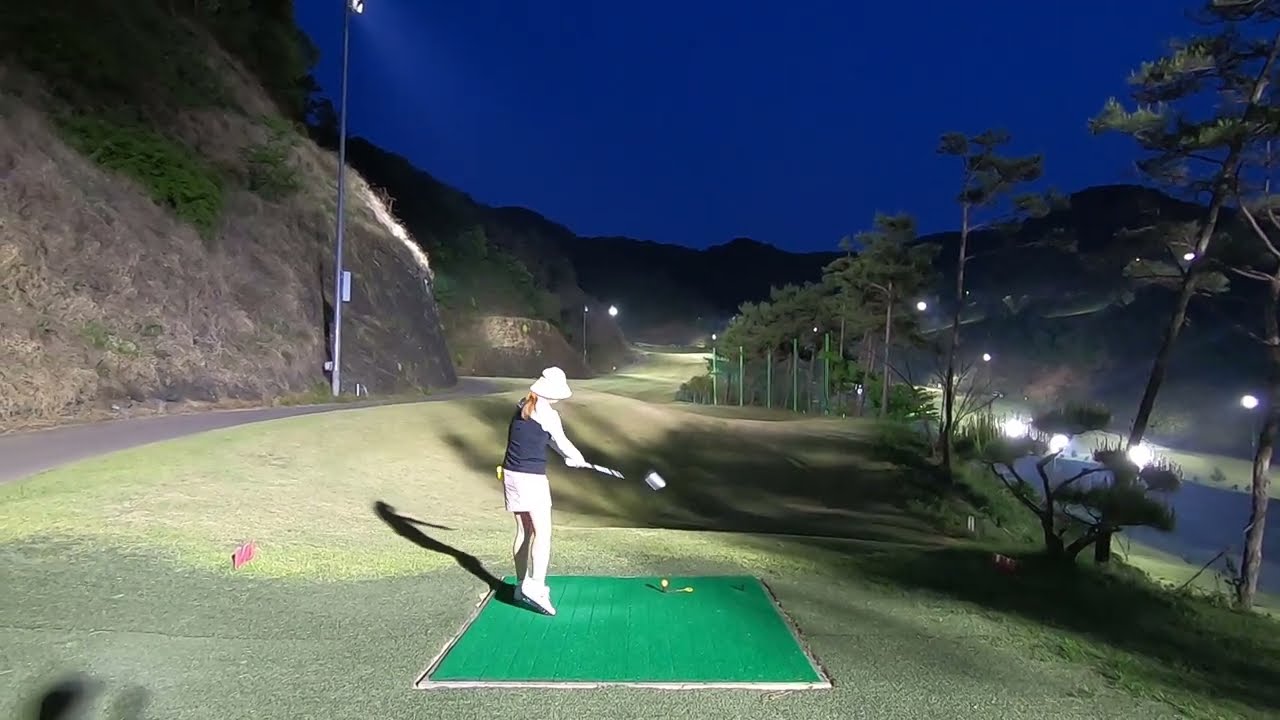The nighttime image captures a woman on a miniature golf course, illuminated by various lights. In the center of the scene, a green rectangular patch features a yellow golf ball. The woman, positioned at this patch, is practicing her swings. She is dressed in a white bucket hat, a blue and white t-shirt, a white short skirt, and white tennis shoes, with her hair pulled back into a ponytail. The surrounding area comprises green artificial grass. To the left, there's a small road or pathway of black asphalt adjacent to a tall cliff or hill. On the right side of the scene, a blue fence with lights directs attention towards the center. The deep blue sky in the background suggests early nighttime, adding to the serene ambiance of the setting.